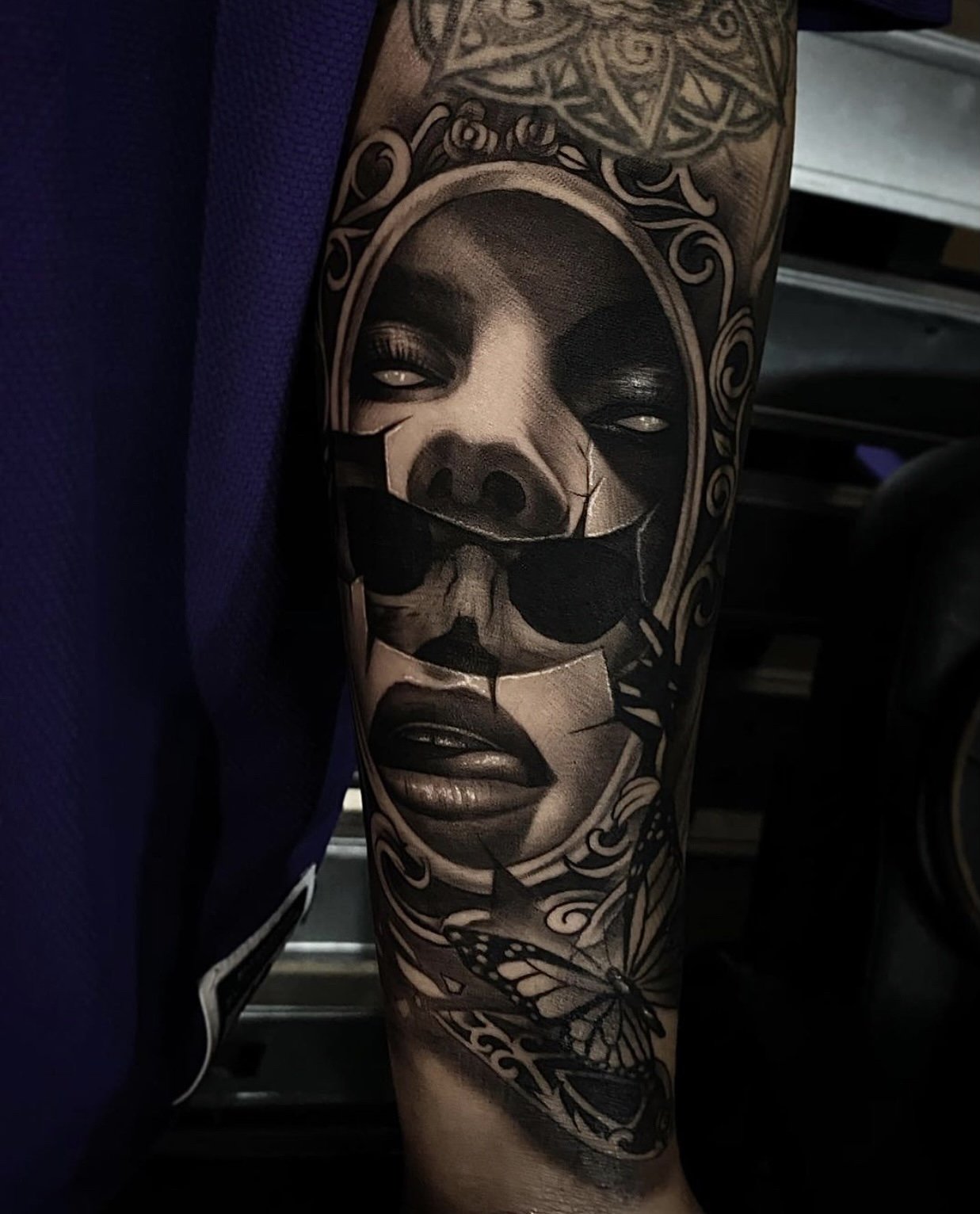This image showcases a detailed, full sleeve tattoo that seems to be inked on the back of a person's arm. The tattoo stretches from the shoulder down, likely to the elbow, and potentially even more. The design is centered around an oval, broken mirror motif, which presents a fragmented depiction of a woman’s face with long eyelashes and white, reflective eyes. The top and bottom fragments of the mirror display distinct facial features, including parted lips with a slightly protruding tongue. The shattered middle section reveals a skull, suggesting a fusion of beauty and mortality. Surrounding the mirror are swirling, floral-like designs and metallic elements, giving the piece a blend of organic and structural aesthetics. Above the mirror, there appears to be a geometric or Celtic-inspired symbol, enhancing the mystical vibe of the tattoo. Below the mirror, a butterfly is depicted, perhaps in the midst of landing. Additionally, some purple fabric, presumably part of the person's shirt, is visible on the left side of the image, adding a hint of color to the otherwise monochromatic composition.